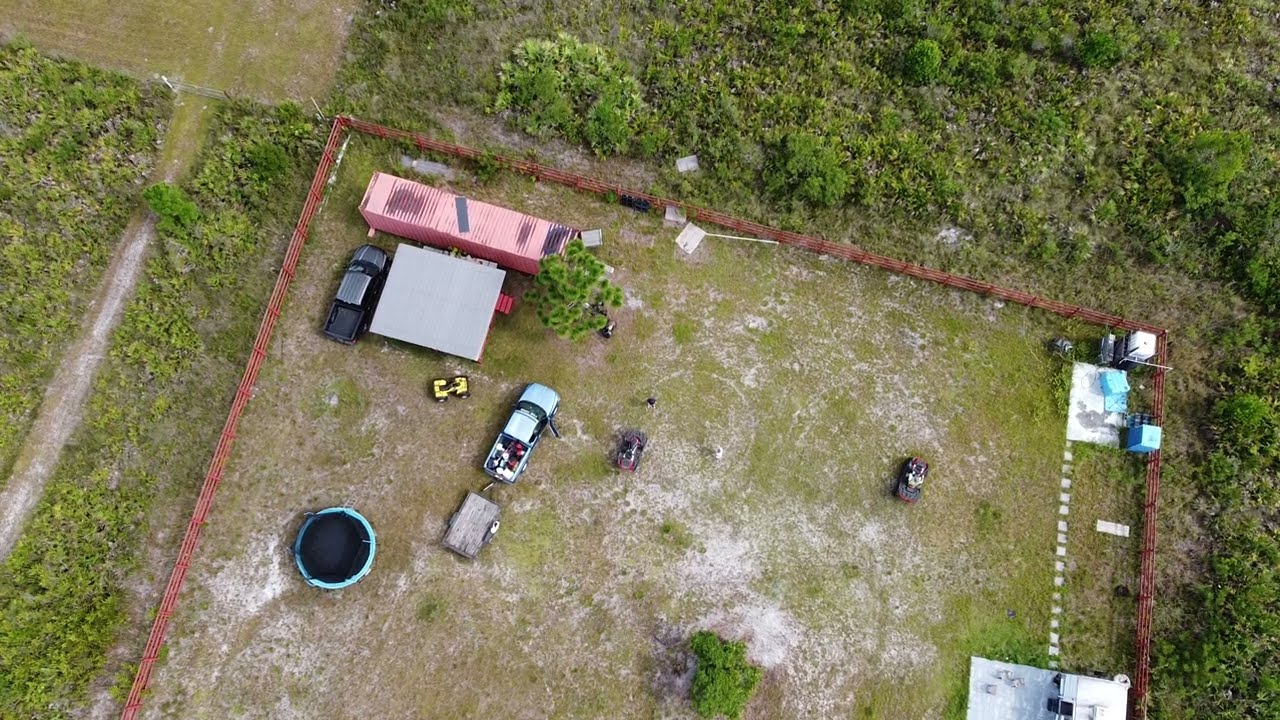This image is an aerial photograph, likely captured by a drone, showcasing a rectangular plot of land encircled by a striking red metal fence, reminiscent of an agricultural barrier designed to keep animals at bay. The ground within the fenced area is characterized by patches of worn grass, exposing a mixture of gray dirt and sandy soil. Positioned towards the upper left of the plot is a prominent pink rectangular container, possibly serving as a storage unit. Adjacent to this container is a gray-roofed structure, under which lies a black pickup truck and a yellow four-wheel ATV. A light blue pickup truck, with its right door open and assorted items in its bed, is hitched to a brown wooden trailer nearby. The fenced area also features a few more scattered ATVs, a big trampoline, a smaller trampoline, and a circular above-ground pool located in the bottom left corner. The boundary of the compound includes what appears to be a stage area. Outside the red fence, the landscape transitions into a mixture of shaggy brush and low green bushes with a dirt road running along the left side, emphasizing the rural, somewhat industrial setting of the compound.